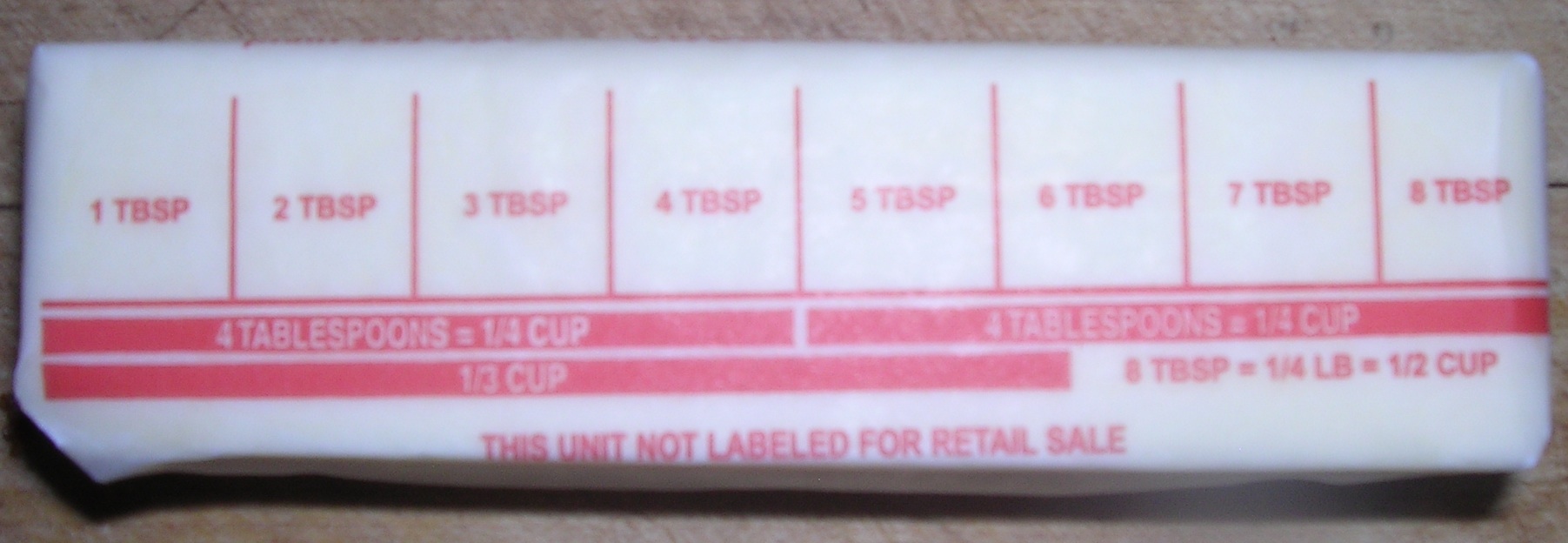A stick of butter, partially covered by its wrapper, is prominently displayed in the image. The wrapper features meticulously marked measurements for precise serving sizes, with a total of eight tablespoons indicated on the stick. Red lines and labels demarcate each tablespoon, from one to eight, while beneath the four-tablespoon mark, additional lines specify that four tablespoons equate to one quarter cup. Another line notes the measurement for one-third cup. Additionally, a label clarifies that eight tablespoons equal one quarter pound, which also equals one quarter cup. Finally, a statement at the bottom of the wrapper asserts that this unit is not labeled for retail sale.